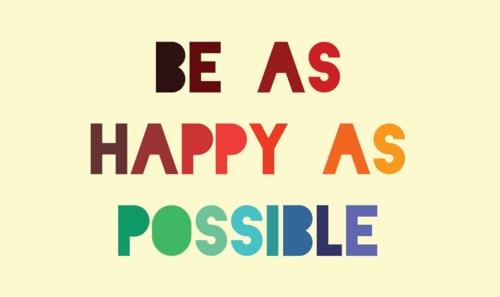The image displays a motivational slogan centered on a pale yellowish ivory background. The text, reading "BE AS HAPPY AS POSSIBLE," is in an all-capital block font with vividly colored letters. The phrase is evenly centered both horizontally and vertically on the background. Each letter is uniquely colored: "BE AS" is in shades of dark red and red-orange, "HAPPY AS" transitions through colors like yellow, green, and blue, while "POSSIBLE" includes even deeper hues such as indigo and purple. This vibrant and cheerful design, possibly created as an art project, evokes a sense of joy and positivity, making it suitable for framing in various settings like an elementary school classroom, a home decor shop, or as a decorative piece in an office or playroom.